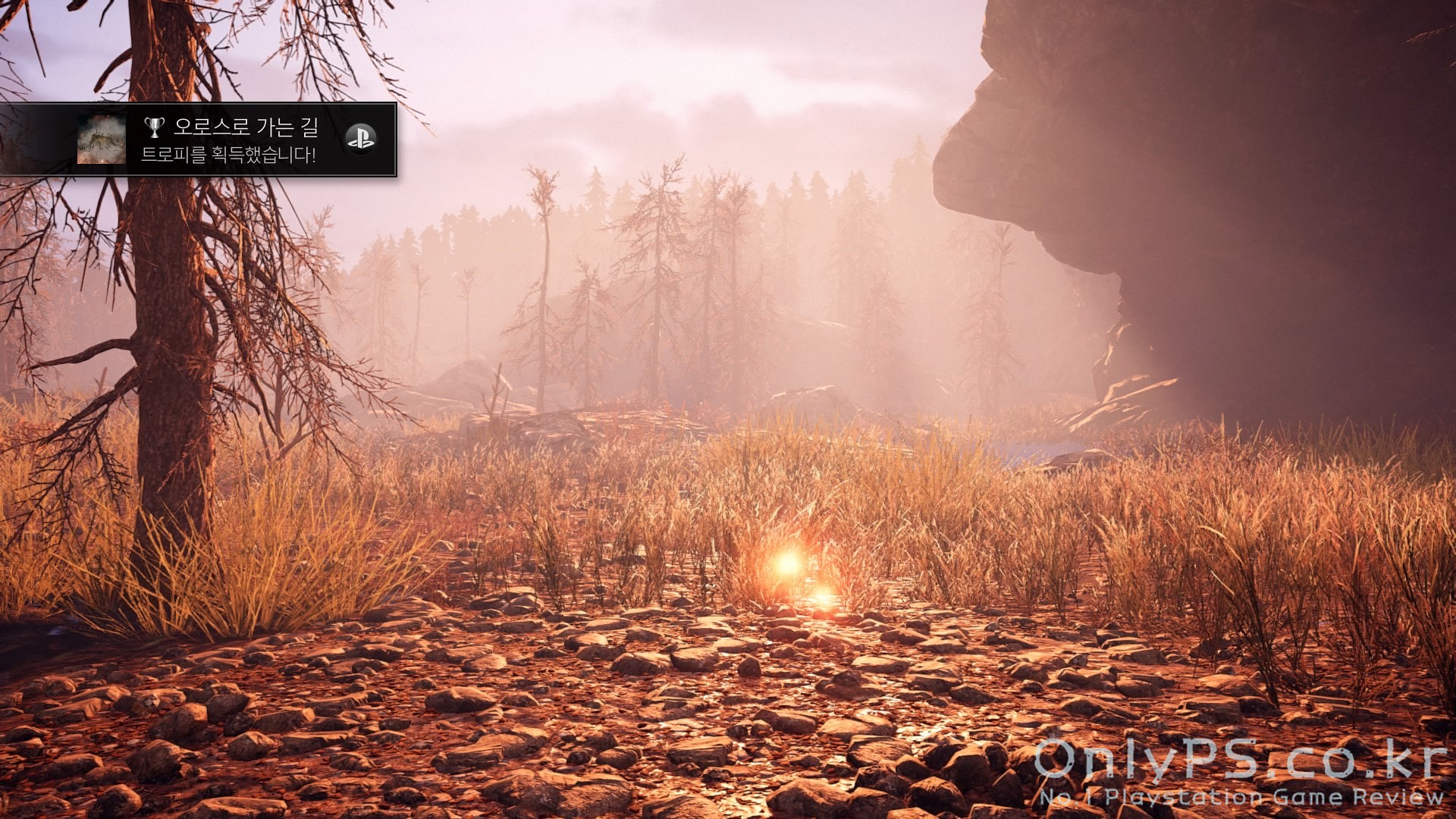The image is a highly detailed, well-rendered screenshot from a video game, displaying a dry, almost fire-ravaged forest scene. The ground is covered with clay-like dirt, scattered rocks, and sparse, brown vegetation. Two round, fiery images dominate the middle of the scene. Large evergreen trees surround the foreground, with healthier trees visible in the background, enveloped by a thick, mysterious haze. A prominent cliff and a dead pine tree, marked with Asian writing on a green rectangle, add to the desolate atmosphere. The sky above is cloudy and foggy, with a bright sun casting a stark light across the landscape. The image features a watermark at the bottom right, reading "ps.co.kr number one PlayStation game review," coupled with a PlayStation logo and trophy icon with Asian characters on a black banner in the top left corner, indicating it is part of a PlayStation game review site.